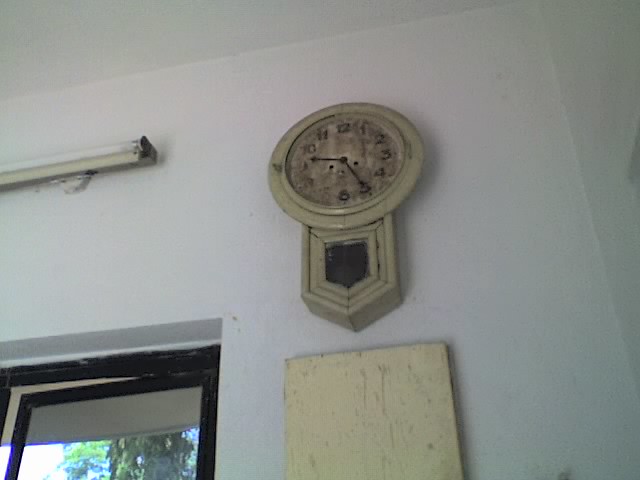This photograph captures an aged, grungy schoolhouse-style clock mounted on a white wall inside a room. The clock is circular with an additional pendulum bottom, reminiscent of a sword with straight lines culminating in a triangular point and a small window for the pendulum. The clock's face, originally white, is now very dirty and features black numbers and hands indicating the time is 9:25. 

In the lower left corner of the image, there is a partially opened window with a black frame, allowing a glimpse of a light sky with some sun, patches of blue, and green trees outside. Also noticeable along the upper left edge of the wall is a large, unlit fluorescent light. Below the clock, a worn, yellowish piece of wood about a foot wide leans against the white wall, further accentuating the room's overall old and neglected appearance.